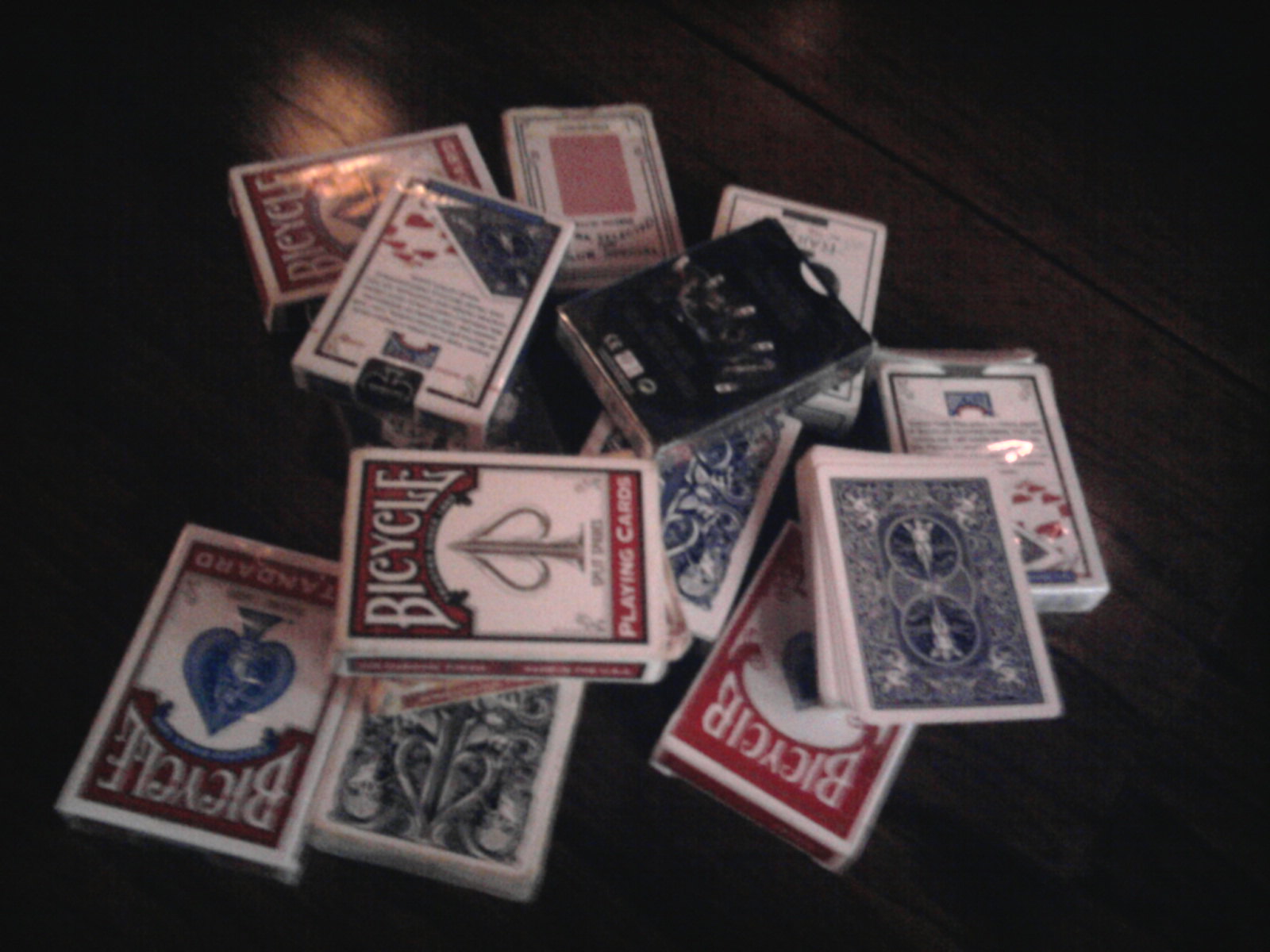The image depicts a chaotic scene of playing cards, with various decks scattered across a dark brown wood table. A total of twelve card boxes are visible, with one of those boxes partially open, revealing a pile of cards atop it. These cards feature a blue design in the center surrounded by a white border. Six of the boxes prominently display the iconic Bicycle brand, characterized by white capital letters on a red background. The text "Playing Cards" is printed at the bottom of these boxes, accompanied by the image of a spade. There is also one black box with an unreadable label and an intricate design. The entire collection of cards and boxes appears to be strewn about in a haphazard manner. Light illuminates the scene from the top left corner, suggesting it's either from a light bulb or sunlight streaming through a window.